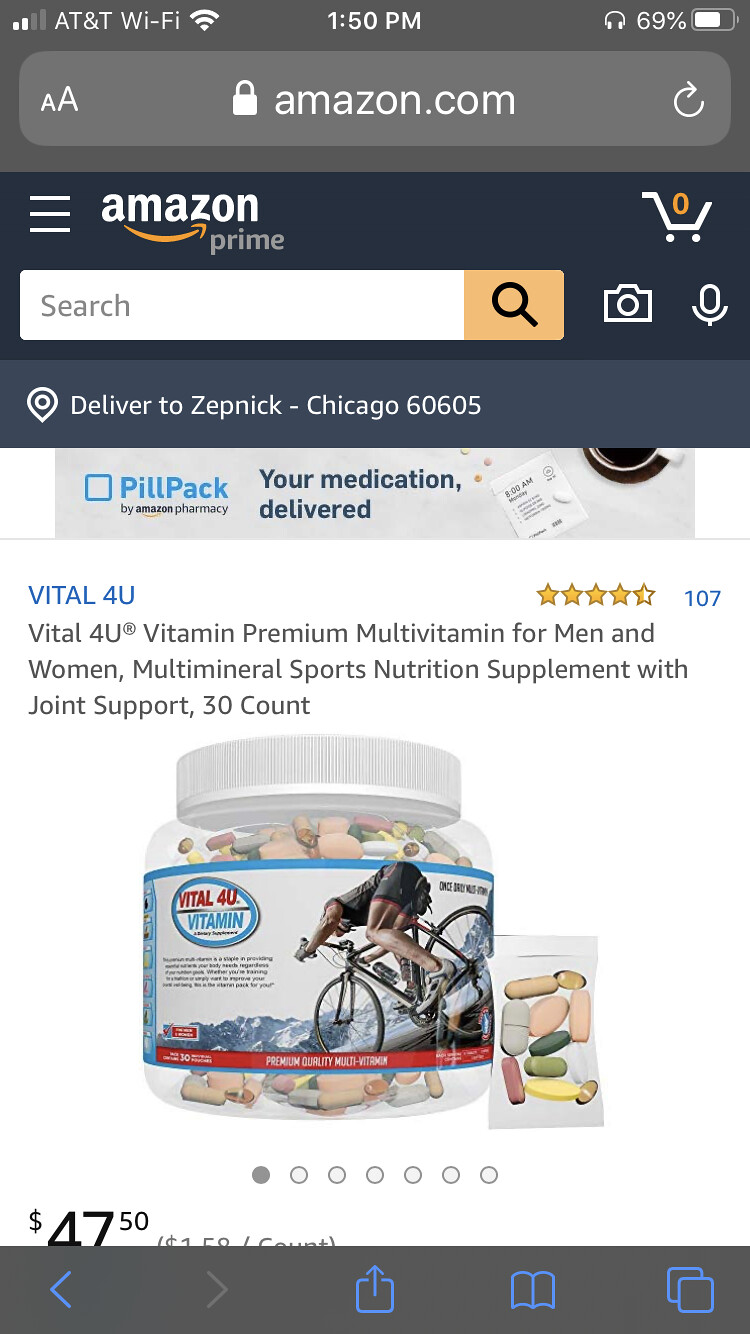A digital recreation of a smartphone screen displaying an Amazon.com product page. The upper third of the image replicates a typical cell phone status bar, featuring the AT&T Wi-Fi logo, the Wi-Fi signal icon, the time "1:50 PM" in white, and the battery icon indicating "69%". 

Below, the Amazon Prime ribbon is clearly visible at the top of the page, with a search bar and a cart icon in the upper right corner. The central focus of this screen is an image of a product—a clear container with a white cap and label. The label, in red, reads "Virtual4U Vitamin", and includes an illustration of a person riding a 10-speed bicycle, depicted from a three-quarter rear profile. 

Adjacent to the container is a clear, rectangular envelope containing approximately seven or eight vitamins, in various colors including tan, white, and clear. 

The product price, "$47.50", is displayed in the lower left corner. At the very bottom of the screen, the black horizontal navigation bar shows icons for navigation, including left and right arrows, a page refresh icon, and a scrolling icon. 

The product description above includes the brand name "Virtual4U" in blue letters, immediately followed by "Virtual4U Vitamin, Premium Multivitamin for Men and Women, Multiple Multi Mineral Sports Nutrition Supplement with Joint Support, 30 Count" in black. In the upper right corner, the product rating is displayed with "5.5 stars" and "107" reviews in blue text nearby.